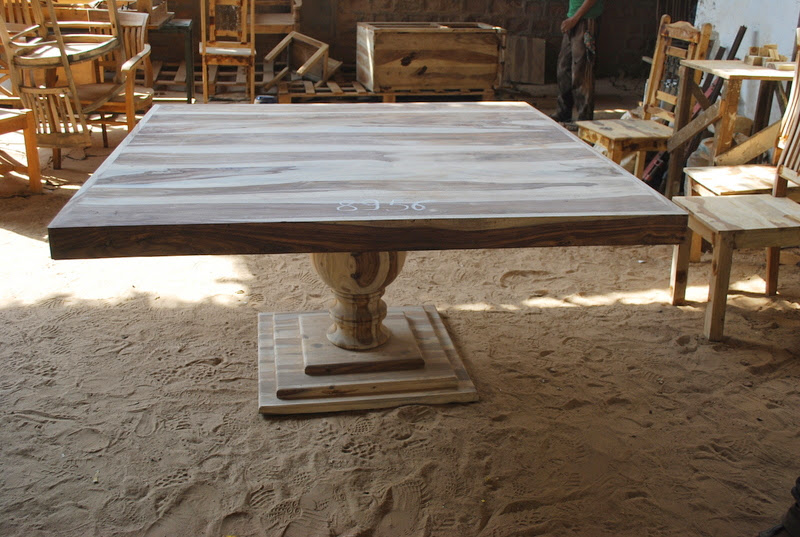The image depicts an outdoor woodworking area with a dominant large, square wooden table. The table stands on a unique base consisting of three descending square platforms and a central roundish pillar. The surface appears sandy, well-trodden with numerous footprints, possibly dirt or sawdust, suggesting it's a heavily used, open-air workshop. Sunlight streams through the scene from the left to the right, casting a glow across the ground. In the background and along the perimeter, numerous wooden chairs and various furniture items are scattered, some stacked or appearing in several states of repair. A man in brown trousers and a green t-shirt walks towards a large wooden box on the right side of the image, reinforcing the element of human activity in this woodworking space.